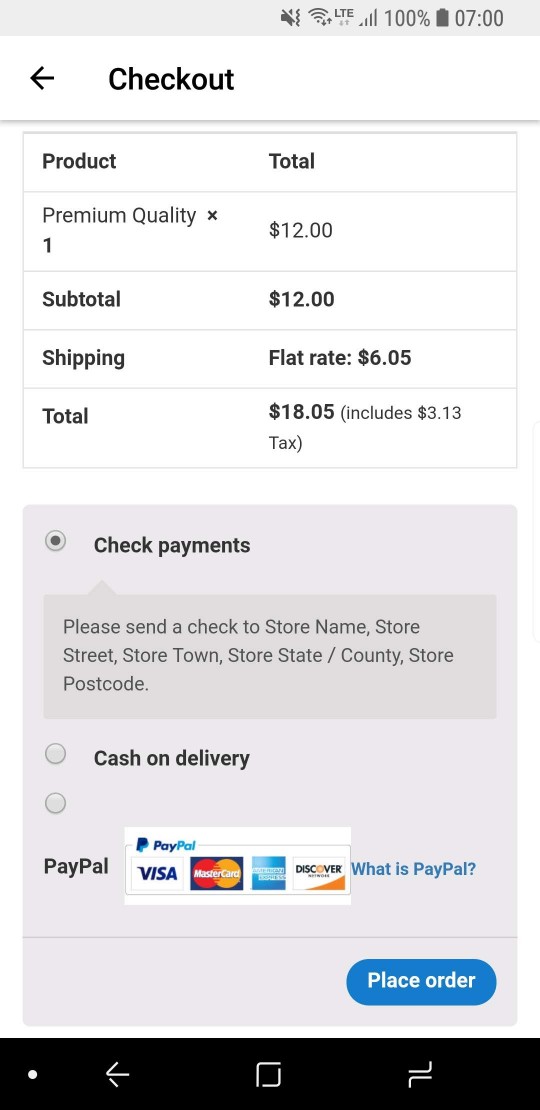A mobile screenshot from an Android device depicting the final steps of an online purchase. The top status bar shows the phone is on silent, connected to full Wi-Fi and LTE, and has a 100% battery at 7 AM.

The checkout page shows the following details:

- **Product:** Premium Quality (Qty: 1) - $12.00
- **Subtotal:** $12.00
- **Shipping:** Flat Rate - $6.05
- **Total:** $18.05 (includes $3.13 tax)

The payment section provides instructions for sending a check to the store, but the placeholder text suggests the setup is incomplete, as it lacks specific mailing information. Other payment options include "Cash on Delivery" and "PayPal," the latter supporting Visa, MasterCard, American Express, and Discover.

At the screen's bottom, a blue rectangular button labeled "Place Order" indicates the final step in completing the purchase.